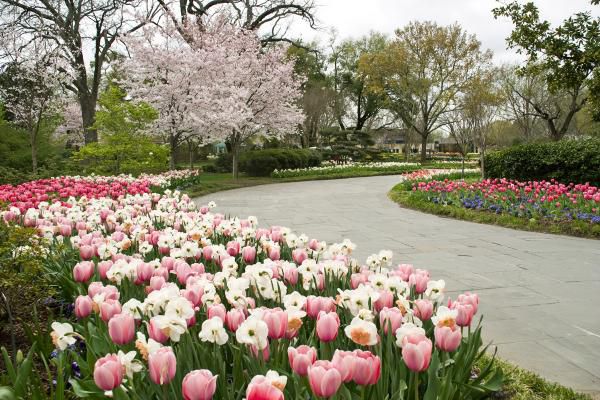The image depicts a beautifully maintained arboretum garden during the spring season. A curved concrete path extends from the lower right corner upward towards the middle of the picture, bordered by a vibrant variety of flowers and trees. On the left side of the path, hundreds of roses in pink hues mix harmoniously with white daffodils, extending towards the background where a large tree in full bloom—possibly a cherry blossom or some type of flowering apple or crabapple tree—takes center stage. The right side of the path is adorned with purple flowers, pinkish-red tulips, and several well-trimmed bushes and trees. The attention to detail and the lush arrangement of flowers, including the striking pink roses and white daffodils following the curve of the pathway, create a picturesque spring garden scene.